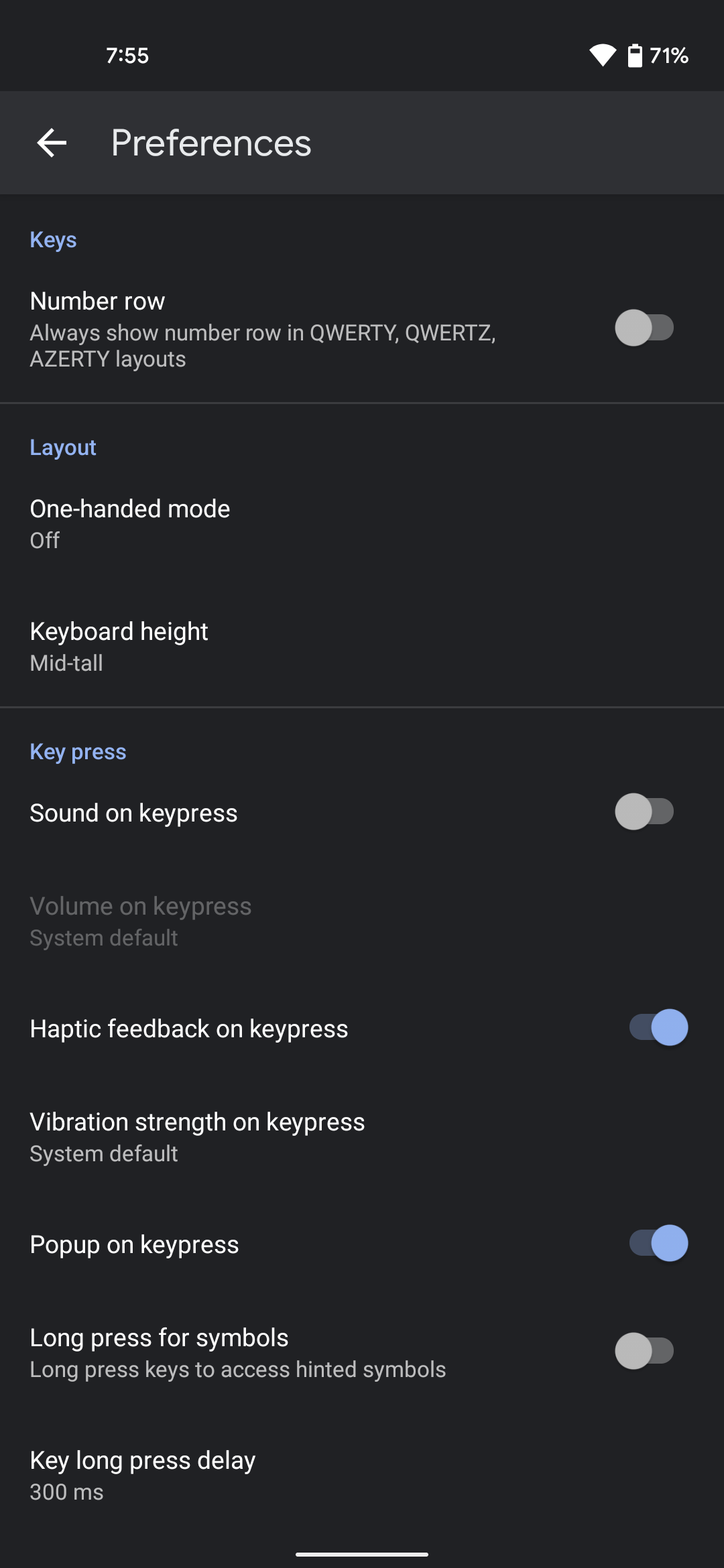This image, captured from a mobile device, displays the user's preferences page, set against a predominantly white background with occasional black elements. Most of the text is displayed in white, with highlights of blue and sections of gray indicating specific options or settings.

At the top of the screen, the status bar indicates the time as 7:55, shows a Wi-Fi connection, and reveals that the battery is at 71% charge. Directly below the status bar, an arrow icon points left, indicating a back option, next to the header labeled "Preferences."

Beneath this header, in blue text, the word "Keys" is prominently displayed. The first option listed under this section is "Number row," with a description explaining that the number row option applies to QWERTY, QWERTZ, and AZERTY layouts. The associated toggle switch for this setting is gray and positioned to the left, signifying that the feature is turned off.

Following a faint gray divider line, the next section labeled "Layout" contains options for "One-handed mode," which is currently disabled, and "Keyboard height," set to "Mid-tall."

Another faint gray separator leads to the "Key press" section outlined in blue text. Here, several options are displayed: "Sound on key press," which is turned off, "Haptic feedback on key press," which is enabled, "Pop-up on key press," also enabled, and "Long press for symbols," which is disabled.

Each setting is clearly displayed with corresponding toggle switches or descriptive text, providing a comprehensive view of the keyboard customization options available to the user.